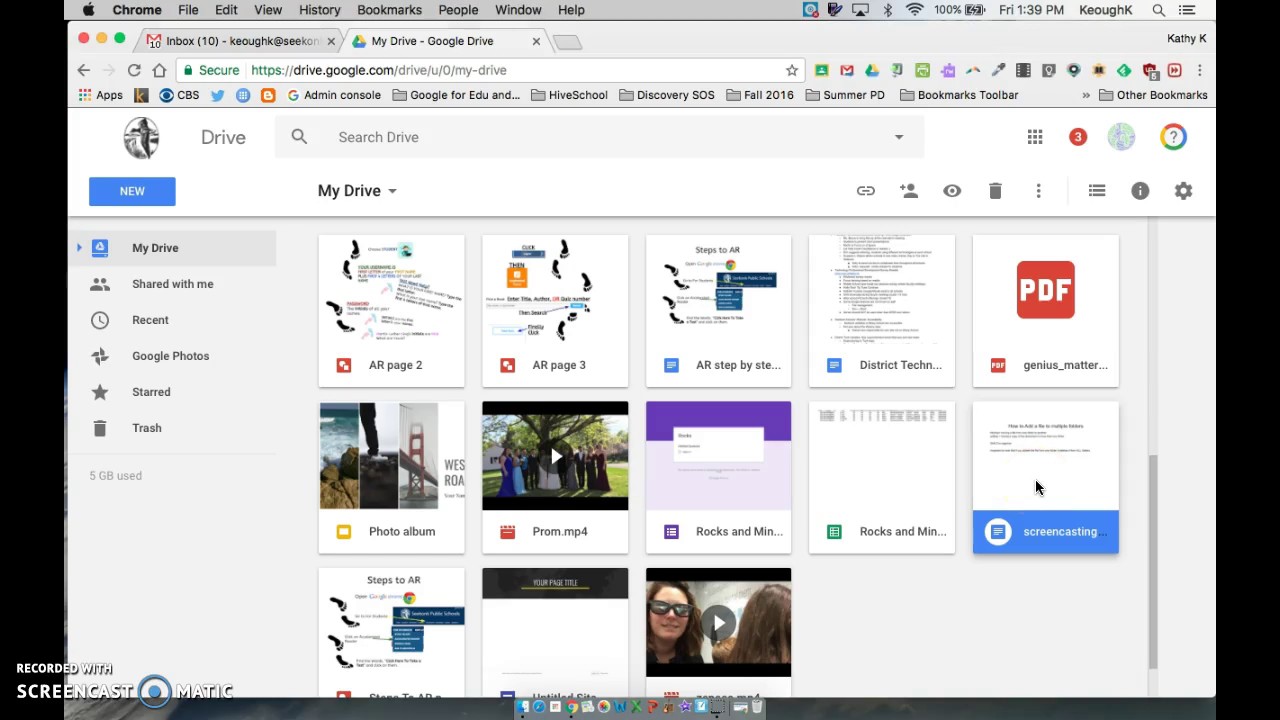This is a detailed desktop screenshot taken during a video recorded with Screencast-O-Matic on an Apple device, showcasing the Google Chrome browser.

At the top of the screen, the Apple menu is visible along with standard Chrome menus: File, Edit, View, History, Bookmarks, People, Window, and Help. The status bar displays various icons including screen sharing, Bluetooth, and Wi-Fi, indicating this is likely a laptop with a fully charged battery (100%). The time is Friday at 1:39 PM, and the user is identified as "Keoughk."

On Chrome, two tabs are open: "Gmail - Inbox" and "S10," with partial email information visible, attributed to Keoughk (or SEKON). Additional Chrome elements include numerous extensions, which appear too small to identify clearly, apart from those for Apps, CBS, Twitter Bookmark, Blogpress, Google for Education, Hive School, Discovery SOS, and seasonal professional development bookmarks.

The main content area displays the user’s Google Drive. The interface shows common Google Drive actions and options such as Drive, Search in Drive, New, My Drive, sharing options, and more settings. The sidebar reveals sections like My Drive, Shared with Me, Recent, Google Photos, Starred, and Trash, indicating 5GB of storage used.

Several documents and files are listed including "AR Page 2," "AR Page 3," "AR Step-by-Step," "District Tech," "Genius_Matter," "Photo Album," "Prom.mp4," and "Rocks and Min" (possibly referring to minerals), along with other unreadable filenames.

Open programs in the Dock include Finder, Chrome, and the Screen Recording Program, while other applications are closed.

Overall, the screenshot captures a detailed view of an individual navigating Google Drive, likely instructing on its features and organization.